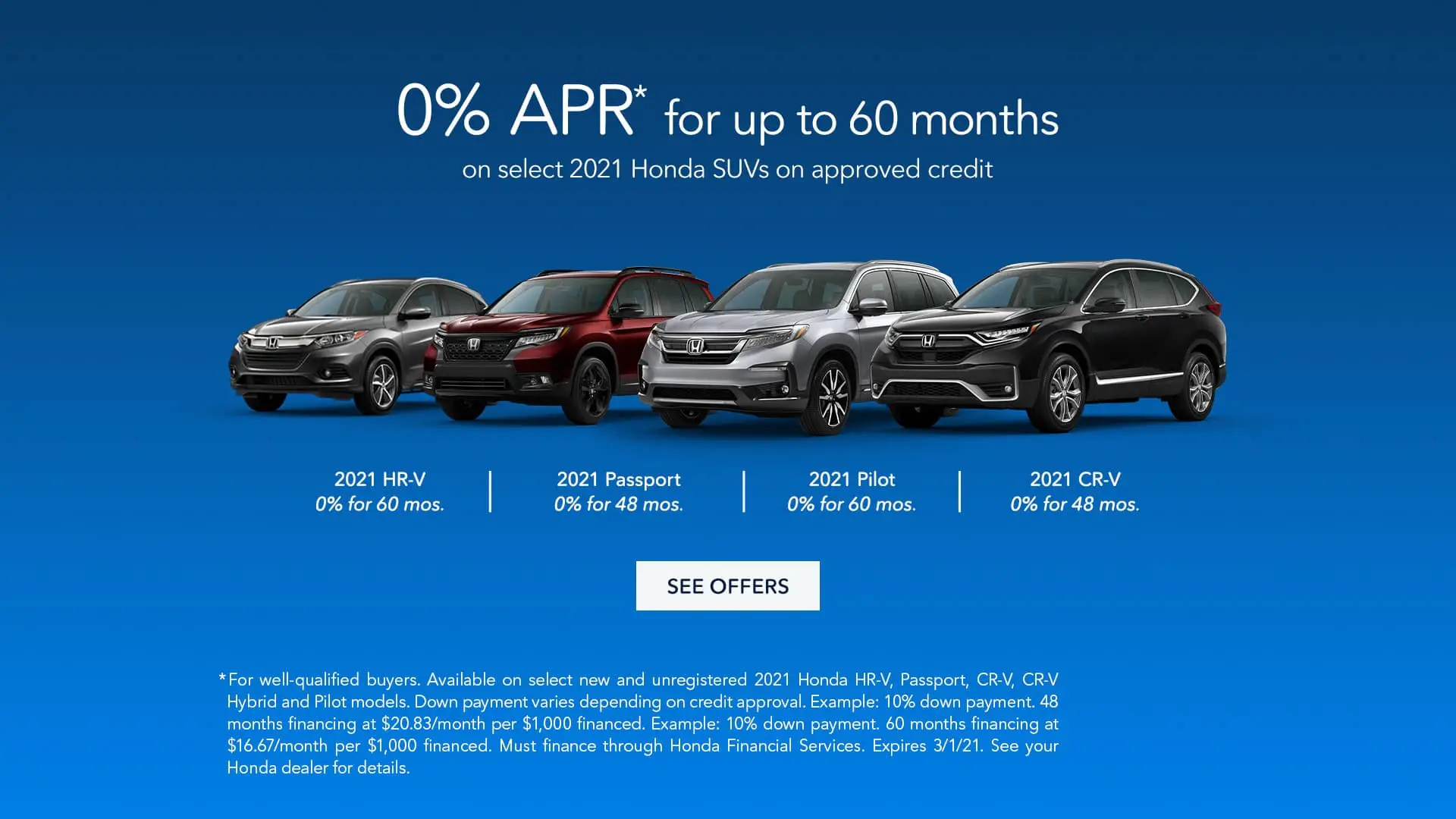The image features a blue background with a gradient transitioning from dark blue at the top to a lighter blue at the bottom. Dominating the center of the image is large, white text reading, "0% APR* for up to 60 months." The "0% APR*" text is the most prominent element on the image. Below this text are four vehicles: a gray 2021 Honda HR-V, a red 2021 Honda Passport, a gray 2021 Honda Pilot, and a black 2021 Honda CR-V. Beneath each car is white text indicating the specific model and year. The image further specifies alternating APR offers beneath the vehicle names: "0% for 60 months" for the HR-V, "0% for 48 months" for the Passport, "0% for 60 months" for the Pilot, and "0% for 48 months" for the CR-V, moving left to right. Centered at the bottom is a white rectangle containing the text "See Offers." Additionally, an asterisk at the bottom middle of the image explains the details of the APR financing, noting that the offer expires on March 1st, 2021.